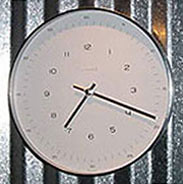This photograph captures a round wall clock with a sleek, thin frame, likely metallic in a dark gray or black color. The clock face is white, featuring bold black numbers and matching black hour and minute hands. It also includes a white second hand that contrasts elegantly against the white background. The clock displays the time as approximately 7:19, with the hour hand just past the 7 and the minute hand near the 4. The wall behind the clock is adorned with vertically striped wallpaper, alternating between metallic silver and black stripes, adding a modern and stylish context to the setting.